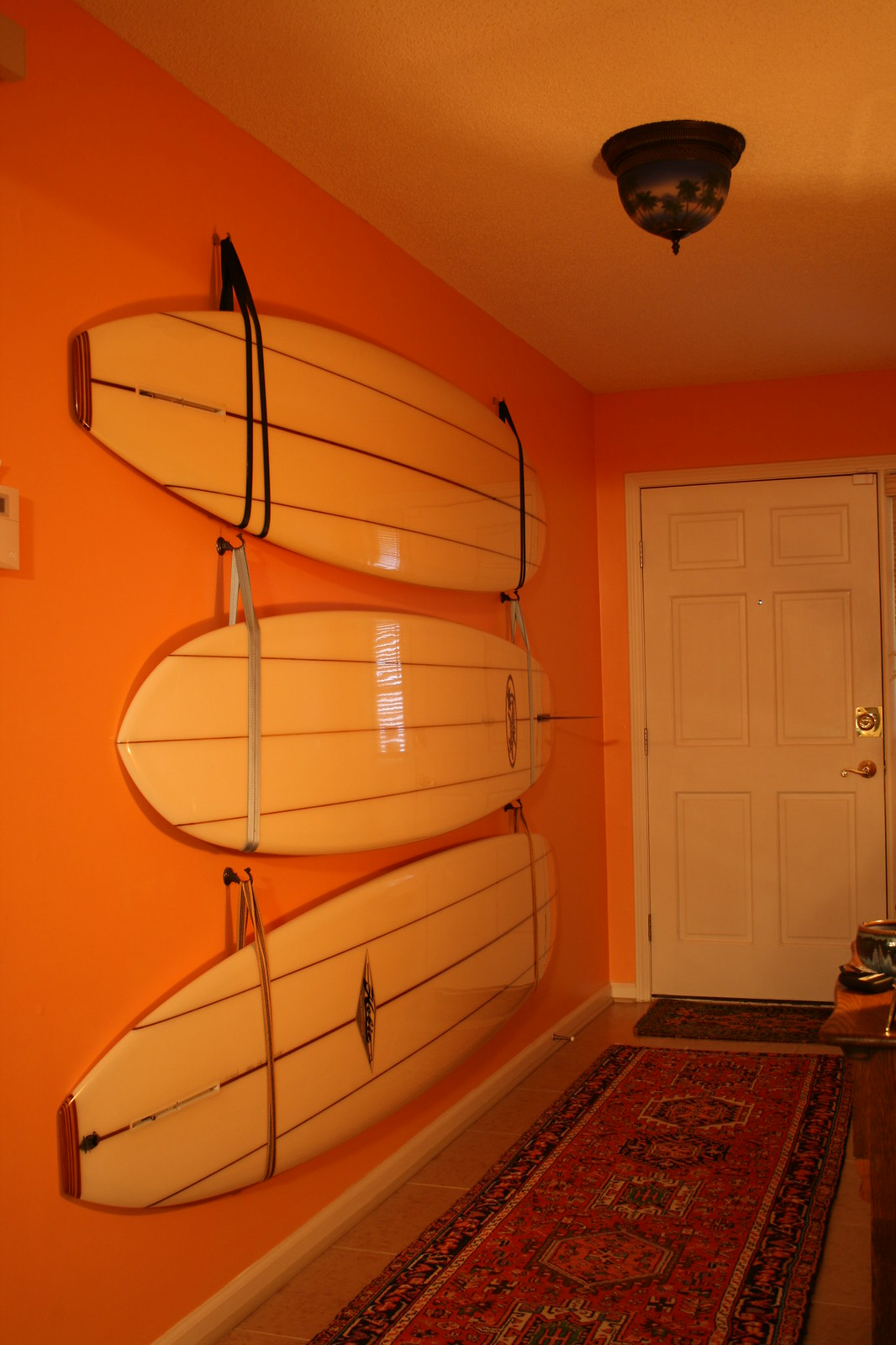This image captures the entryway of a home, featuring a decoratively arranged wall of three horizontally mounted surfboards. The surfboards, each a tannish color with three dark brown horizontal lines, are fastened to an orange-peachish colored wall using black, silver, and yellow striped straps. The surfboards vary in length, with the middle one sporting a visible fin. The entryway additionally showcases a white front door, complete with a golden-colored handle and a deadbolt lock, which opens to the left. Above, a ceiling of undetermined color (due to dim lighting) accommodates a round black ceiling light fixture. The floor is adorned with a Moroccan, mosaic-like rectangular rug showcasing vibrant reds, yellows, blues, and browns, set against light brown floor tiles. To the right, a bench sits ready to hold keys and other small items, rounding out this warmly illuminated and eclectic entryway.